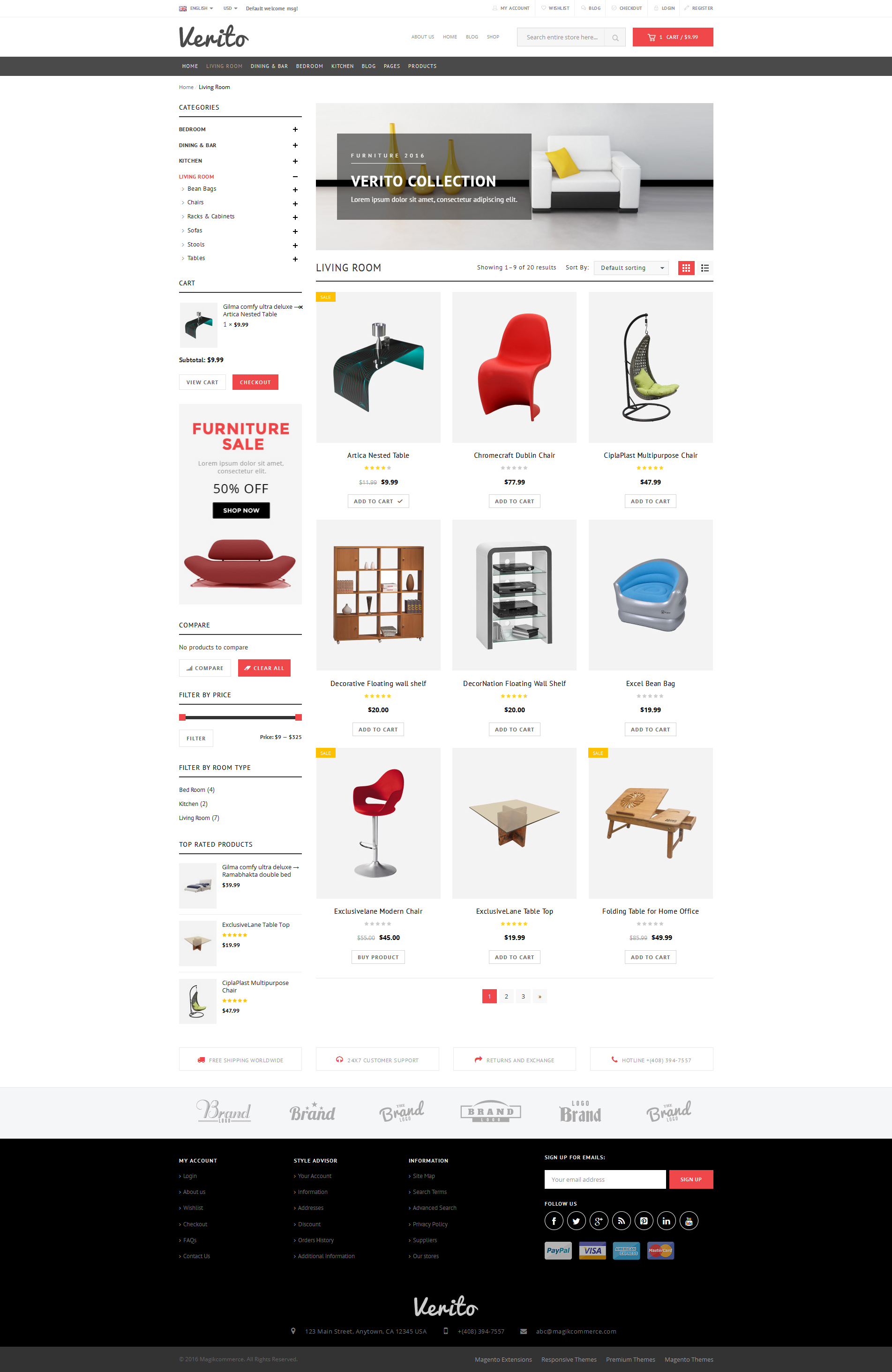**Descriptive Caption of the Verito Website Homepage**

The Verito website, a furniture-centric platform, is presented with a minimalist white background. At the very top left, the Verito logo is prominently displayed. Directly above the logo, users can select their country, language, and preferred currency, with the default set to USD. Adjacent to these options, a welcome message is displayed that reads "Default Welcome Message." 

To the top right of the page, there is a navigation menu including options such as "My Account," "Wishlist," "Blog," "Checkout," "Login," and "Register." Beneath this menu, another set of links like "About Us," "Home," "Blog," and "Shop" is present, along with a search bar and a red cart icon indicating one item in the cart priced at $39.99.

The left sidebar showcases various categories including "Bedroom," "Dining & Bar," "Kitchen," and "Living Room." The "Living Room" category is expanded to reveal sub-categories such as beanbags, chairs, racks and cabinets, sofas, stools, and tables. Within the small cart window, a "Gilma Comfy Ultra Deluxe Artica Nested Table" is added to the cart either priced at $39.99 or $9.99.

A banner promoting a "50% Off Furniture Sale" with a prompt to "Shop Now" is visible next. Below the banner are "Compare" and "Filter" tabs, with the filtering option allowing users to sort by room type. A list of top-rated products is also available.

On the right-hand side of the homepage, the "Living Room" category is highlighted in bold black text, showcasing a variety of furniture items. These include the "Artica Nested Table," "Comcast Dublin Chair in Red," "Siplaplast Multi-Purpose Chair," a decorative shelf, wall shelf, Excel beanbag, a modern chair, tabletop fixtures, and a floating work-from-home table.

Towards the bottom of the page, various brands are listed, followed by a "My Account" menu offering several options for user management. Additionally, a "Style Advisor" section provides personalized style advice, and an "Information" menu delivers essential details about the site. A small email signup box sits on the right side, accompanied by links to Verito's social media profiles.

Overall, the website is well-organized, providing a thorough and structured browsing experience for furniture enthusiasts.